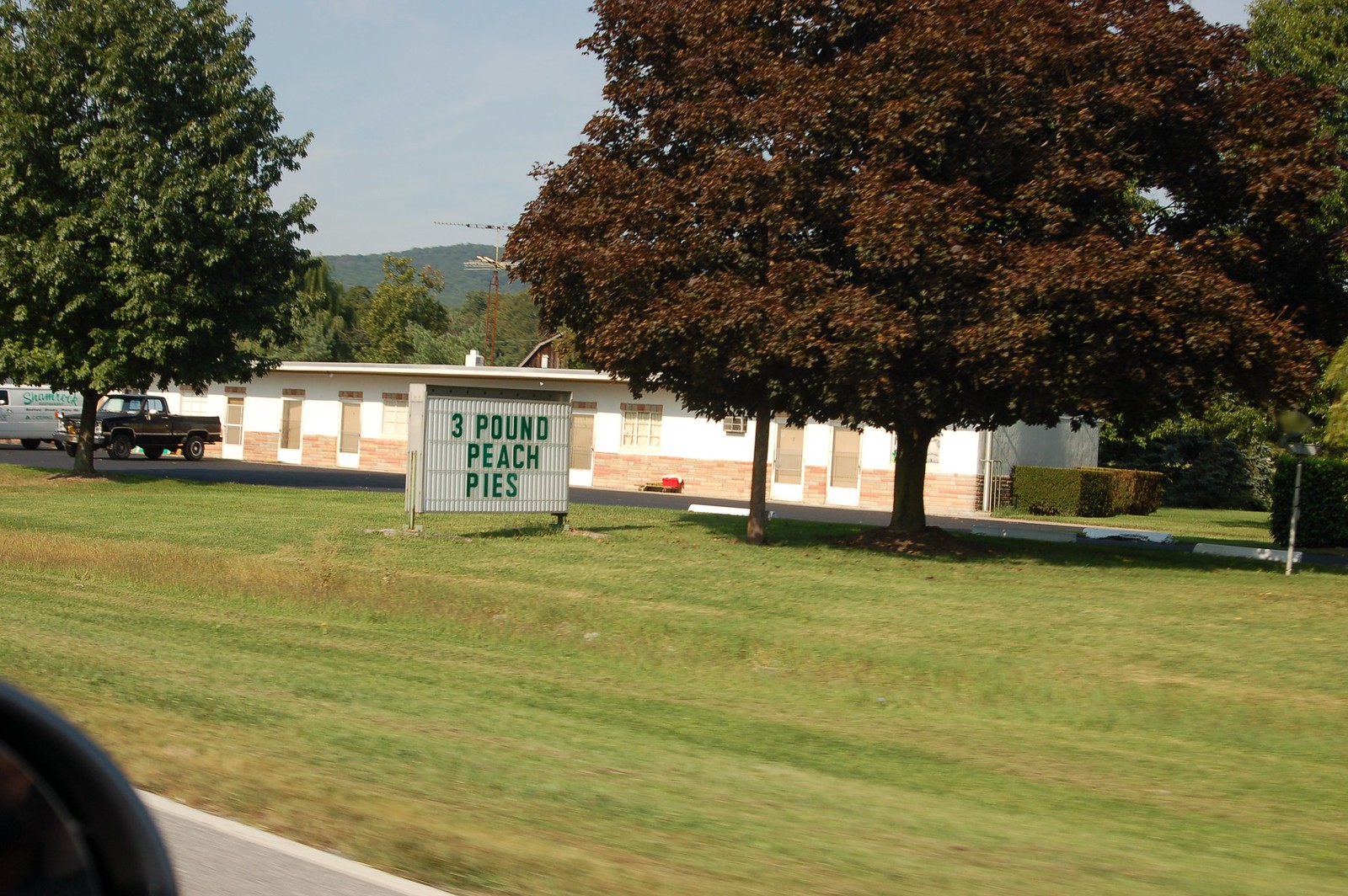The image depicts a view from a car window, as evidenced by the edge of the rearview mirror in the lower left corner. The scene primarily shows a well-maintained grassy field with a few dirt patches. To the left, there's a green-leaved tree, while to the right, we see trees with reddish leaves and a green and red bush next to a white sign that reads "Three Pound Peach Pies." In the foreground, a black pickup truck and a partially visible white van with green writing, potentially saying "Shamrock," are parked. Dominating the mid-ground is a long, rectangular, one-story building with a white top and reddish brick bottom, featuring several doors and windows. Additionally, in the backdrop, tall trees reach to the top of the photo, with a mountaintop and possibly a crane visible in the distance.